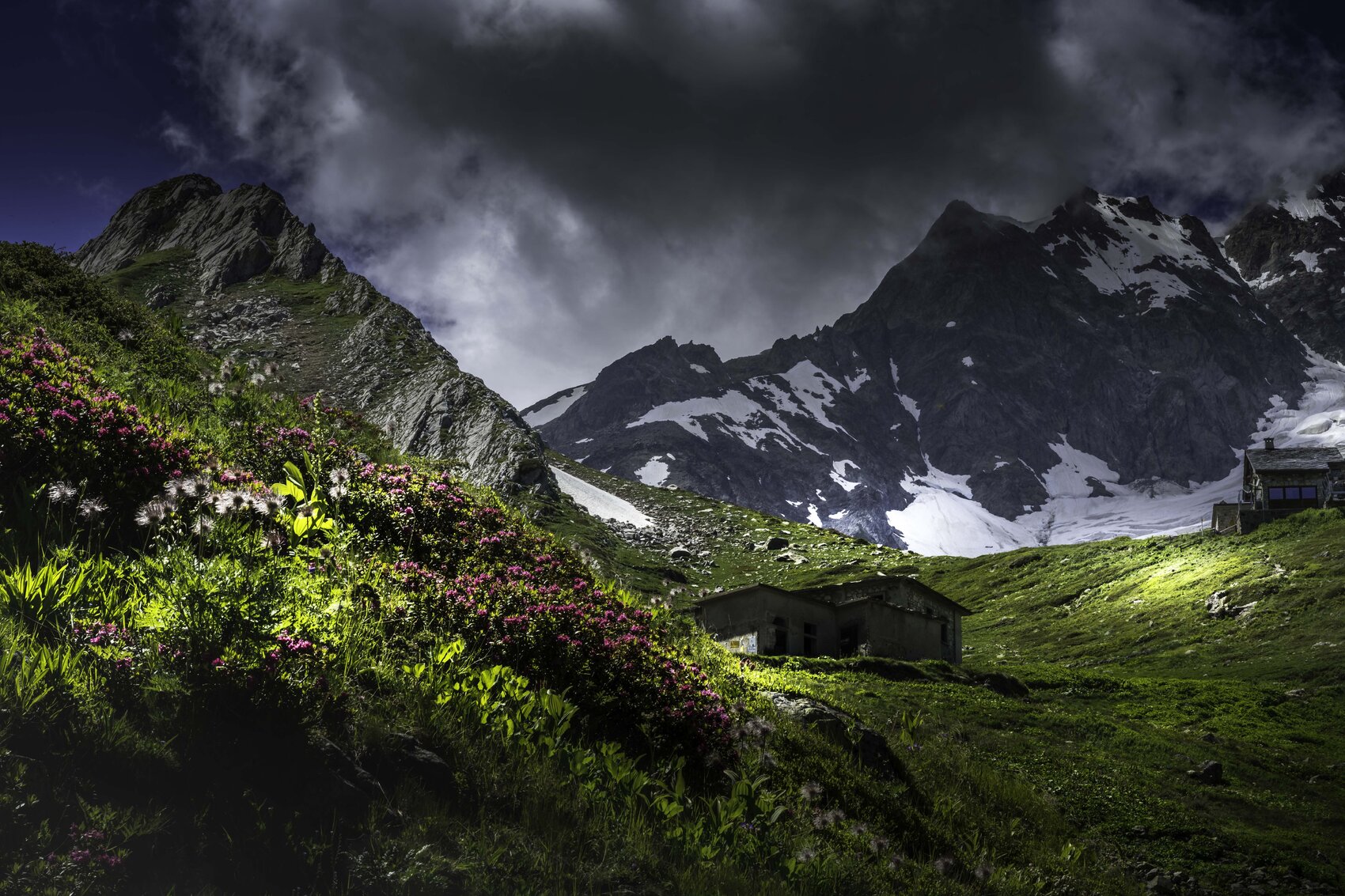In this captivating alpine landscape photograph, a quaint, classic two-roof cottage sits slightly off-center amidst a vibrant green valley. The foreground is adorned with lush greenery and scattered wildflowers in hues of purple and white, set against a backdrop of majestic, jagged mountains partially draped in snow. The mountains' dark, stone-gray peaks reach into the sky, which is heavy with dark blue, gray, and white clouds, hinting at impending rain. Fleeting slivers of sunlight pierce through the cloudy sky, gently illuminating patches of the verdant grass around the house. To the right, partially framed by the snowy mountain, is a Bavarian-style structure, only partially visible. The scene exudes a serene yet somewhat foreboding beauty, with its remote and tranquil setting under the brooding sky.